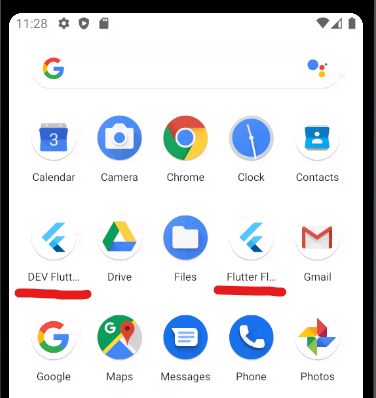This image captures a detailed screenshot of an individual's smartphone home screen. In the upper left-hand corner, the time reads 11:28, accompanied by symbols for Settings, Play, and an SD card. Near the upper right-hand corner, indicators show full Wi-Fi signal, half-full cellular service, and a fully charged battery.

Just beneath these indicators, there's a Google search bar prominently displayed. Below the search bar, a grid of app icons starts from the upper left as follows: Calendar, Camera, Chrome, Clock, and Contacts. The next row contains apps labeled DEV and Flood, with the latter partially cut off and highlighted by a red underline. Further down are the Drive, Files, and Flutter apps, followed by an app abbreviated as Fi or Fl, also underlined in red, and then Gmail.

The subsequent row showcases Google, Maps, Messages, Phone, and Photos apps. Encircling the whole screen, there is a thin black border running along the left, right, and top edges, giving the impression of a framed display.